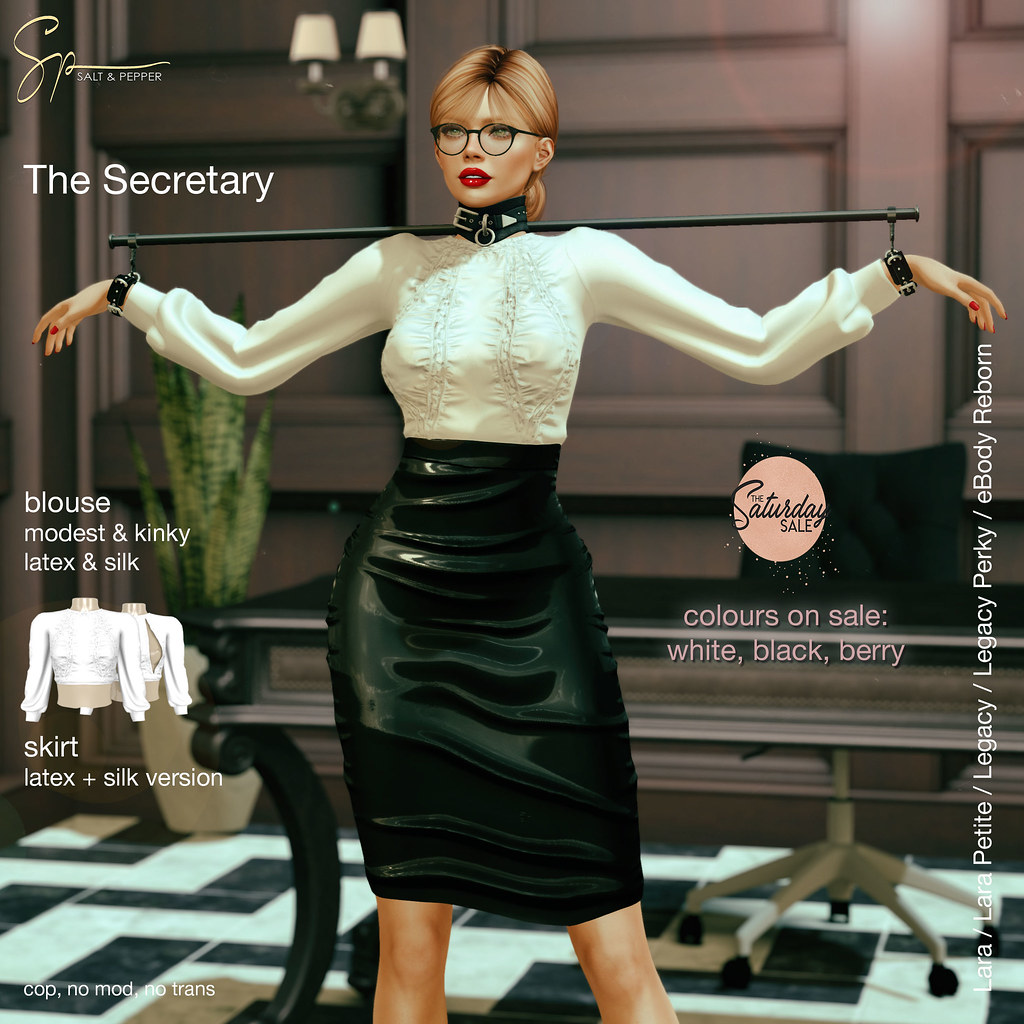This is a square image depicting a 3D-rendered digital character, central to the frame. The character is a white woman visible from the knees upwards, with blonde hair styled in a ponytail and bangs, wearing black glasses and red lipstick. She is dressed in a long-sleeved white silk blouse and a long black leather pencil skirt. Her arms are extended out to her sides, restrained by a long black pole connected from a black collar around her neck to two black bracelets on her wrists, giving a dominatrix-like appearance. She has red nail polish on her fingers.

On the top left of the image, there is a logo in gold that reads "Salt and Pepper." Below it, in white font, it says "The Secretary," possibly referencing the movie "The Secretary." Further down, the text reads "Blouse, modest and kinky, latex and silk skirt, latex + silk version." On the right side of the image, another logo states "The Saturday Sale" with the note "colors on sale: white, black, berry."

The background is a simple setup featuring a black and white stone floor, with some plants and a few lamps.